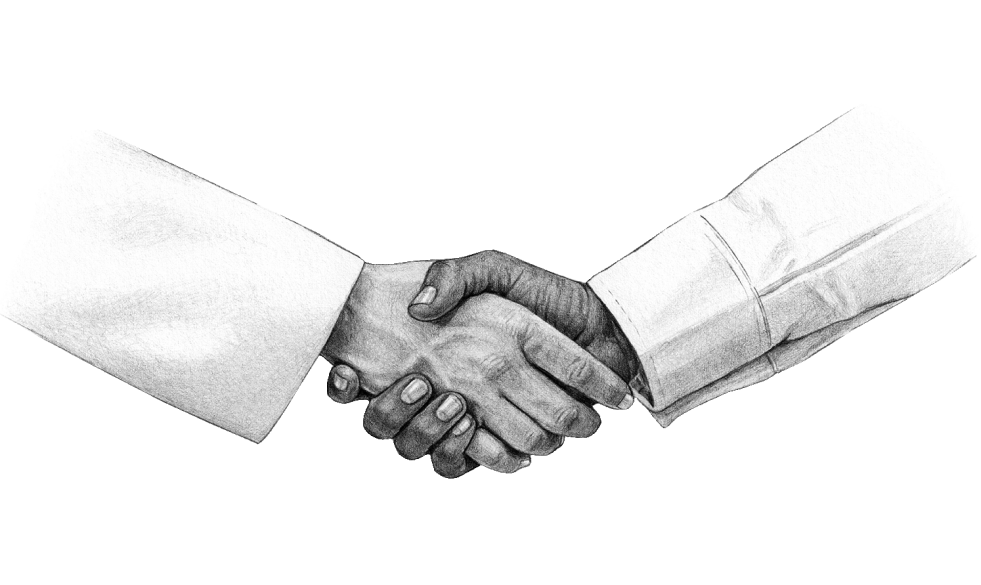This highly detailed pencil or ink drawing features a powerful depiction of two men shaking hands, symbolizing unity and racial harmony. Set against a stark white background, the composition zooms in to display only the sleeves and hands of the two individuals, capturing them from just below the elbow. The intricate rendering shows one hand extending from the upper left corner, with the palm facing forward, grasping another hand from the upper right corner, whose palm is directed towards the viewer.

Both men wear white shirts, but the sleeve on the left has a noticeable cuff around the wrist, while the sleeve on the right does not. The hand on the left appears to belong to a Caucasian individual, while the hand on the right seems to have African American skin. The drawing's rich detail exquisitely portrays veins, creases, knuckles, and nails, bringing a sense of realism and depth to the image. The meticulous shading and clean lines enhance the lifelike texture and highlight the careful attention paid to every nuance of the hands.